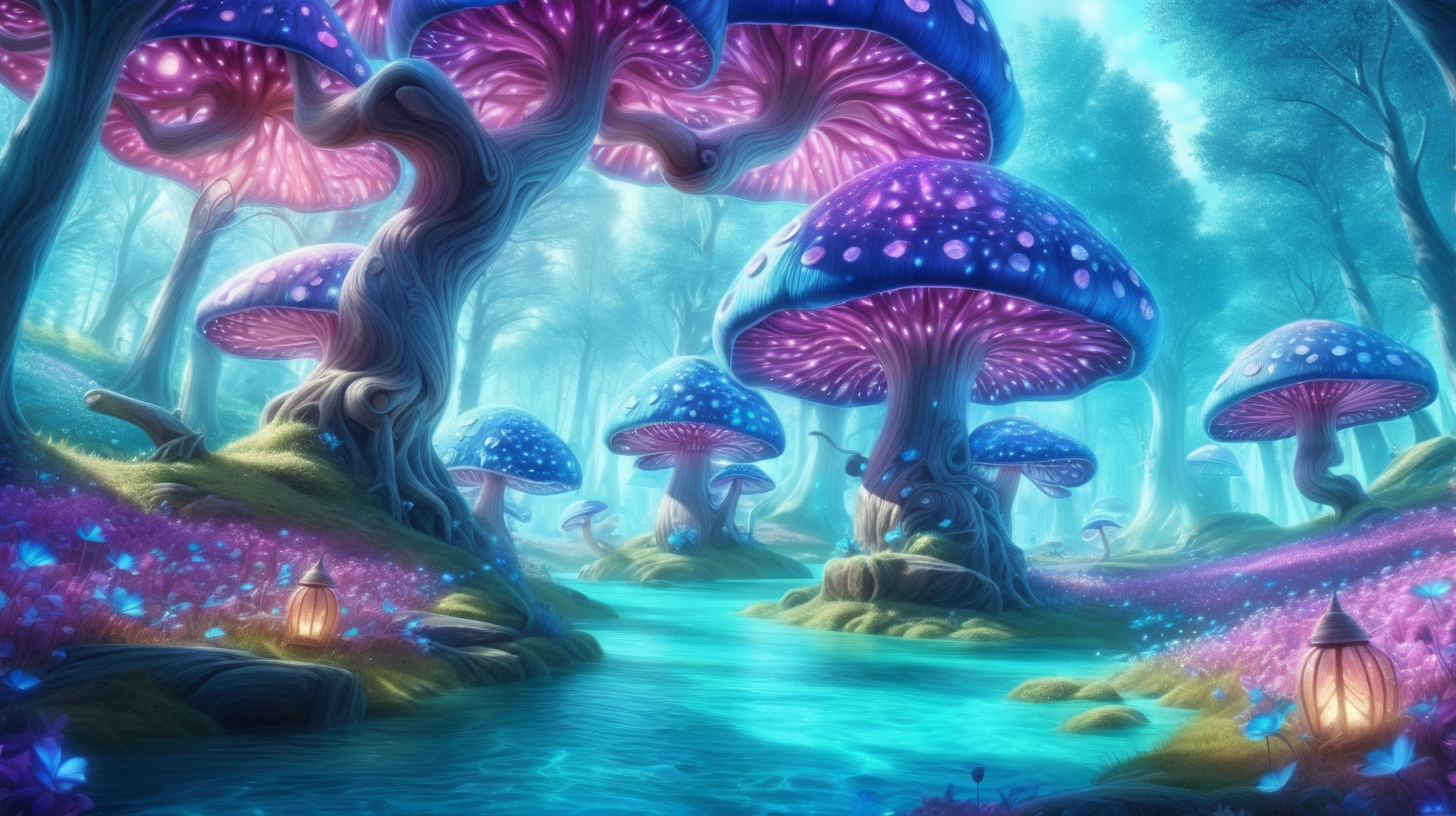This is a stunning 3D graphical AI-illustrated image that vividly portrays a fantastical forest landscape reminiscent of Alice in Wonderland. In this enchanting scene, the forest is dominated by gigantic mushroom trees with massive, tree-like bases and branching offshoots. The mushrooms are a vibrant mix of pink and blue-purple hues, with intricate, glowing lights under their caps. Among them, there are both large and smaller mushrooms, creating a highly detailed and layered composition. The ground beneath features lush green grass, scattered with pink and purple flowers, and accents of blue butterflies fluttering around. A serene lake or river flows gracefully through the scene, reflecting the ambient colors. Towering trees form the backdrop, and a luminous white sky can be seen peeking through the dense foliage, casting gentle light over the entire ethereal setting.